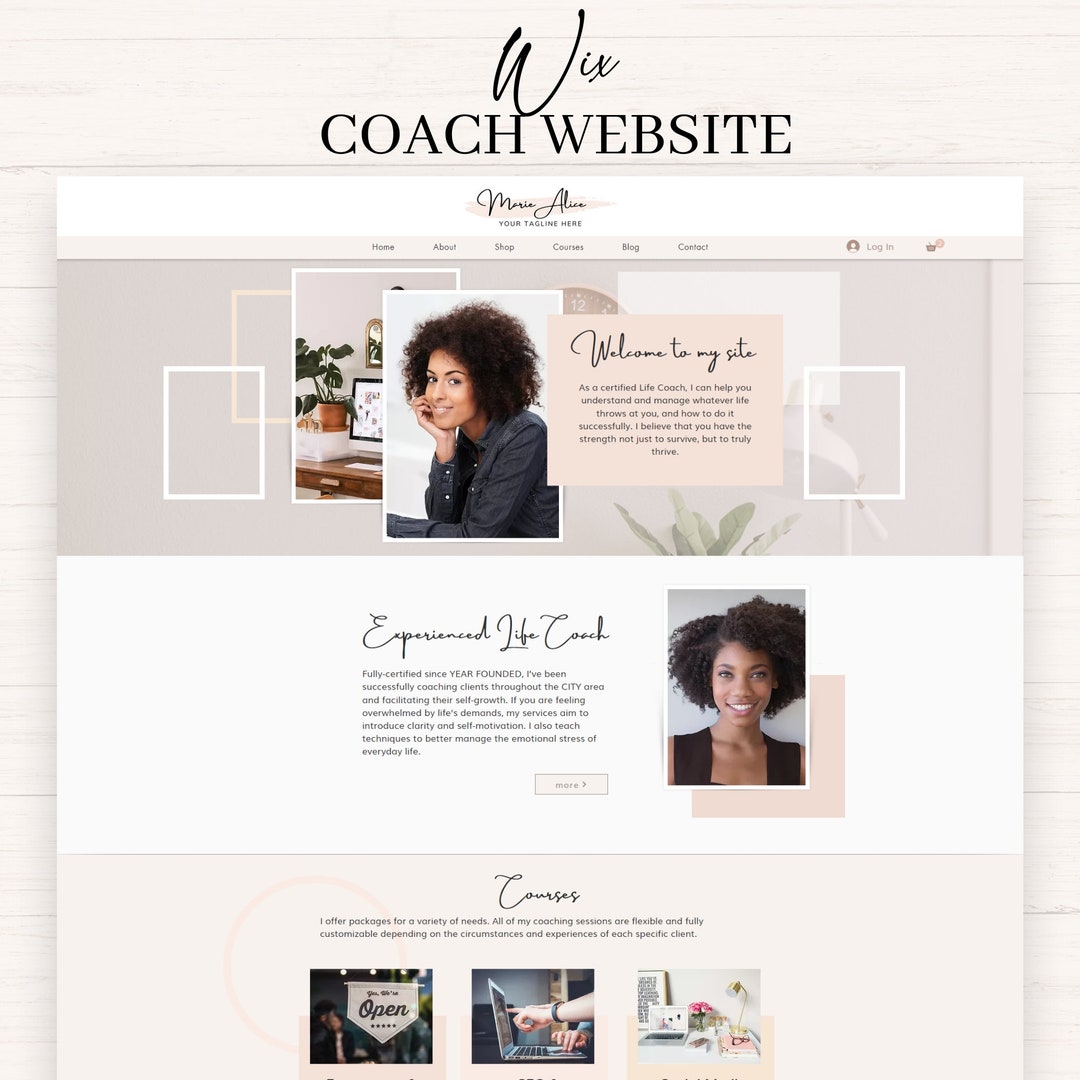The image depicts an advertisement for a coaching service with a modern and stylish website design. At the top of the page, the words "Coach Website" are prominently displayed in black text, accompanied by a distinct "W" symbol above it. Below, there's a visually captivating signature set against a pink background, flanked by navigation categories—Home, About, Shop, Courses, Blog, and Contact—in small yet readable text.

In the next section, a side-view photograph of the coach, who has curly dark brown hair, a slightly darker skin tone, and is wearing a black jacket, is positioned against a light purple background. Adjacent to the image is a welcoming message in cursive, "Welcome to my site," rendered in a pinkish-purple hue, accompanied by a paragraph of black text providing additional information.

The middle part of the page features a white background with the phrase "Experienced Life Coach" elegantly written in cursive. Below it is a front-view image of the coach, along with a descriptive paragraph about their experience and qualifications.

Further down, the "Courses" section highlights three offerings, each represented by a distinct image. This section includes two introductory sentences and is set against a light gray background, consistent with the website's contemporary and sleek aesthetic. The entire layout, including the left, right, and very top of the website, showcases a modern design, making it visually appealing and easy to navigate.